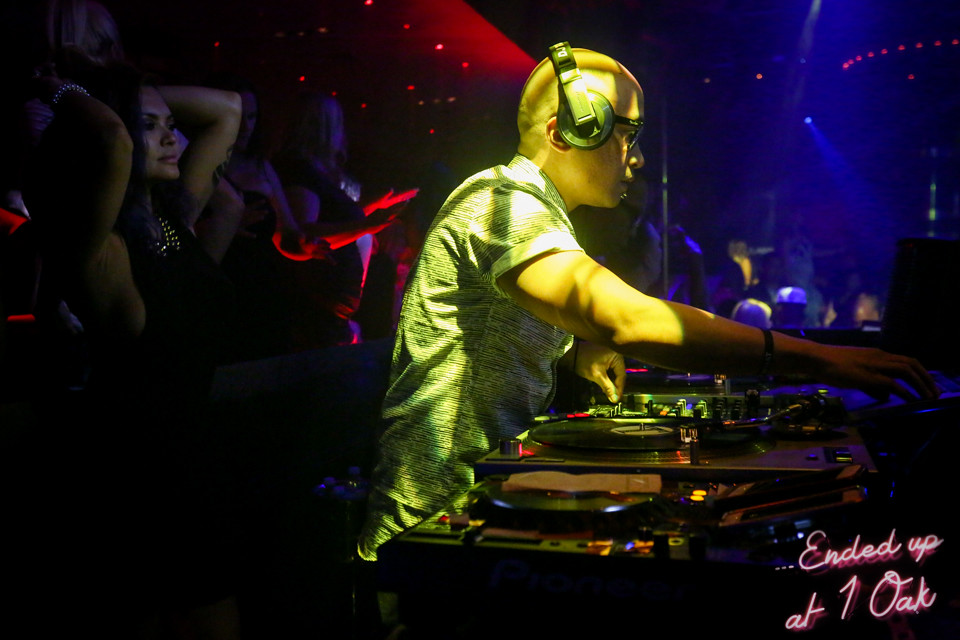The photograph captures a lively scene at a nightclub, with a DJ at the center of attention, bathed in a yellow spotlight. He's wearing a short-sleeved yellow or possibly white shirt with dark stripes and is equipped with wireless headphones and glasses, with a notable piercing on his face. The DJ is actively engaging with his equipment, which includes two turntables and a mix of dials and knobs, alongside a laptop, branded with the word "Pioneer." The backdrop features a dark, smoky atmosphere illuminated by scattered red and blue lights. 

Behind the DJ, a young woman in a black dress with gold accessories has her hands raised, dancing energetically. Additional silhouetted figures can be seen dancing in the distance, adding to the festive mood of the image. Located in the lower right corner, the caption "ended up at One Oak" (O-A-K) is prominently displayed in white text with a pink shadow, anchoring the setting in the iconic club. The overall composition highlights the dynamic interplay of light and darkness, capturing the essence of a vibrant nightlife scene.